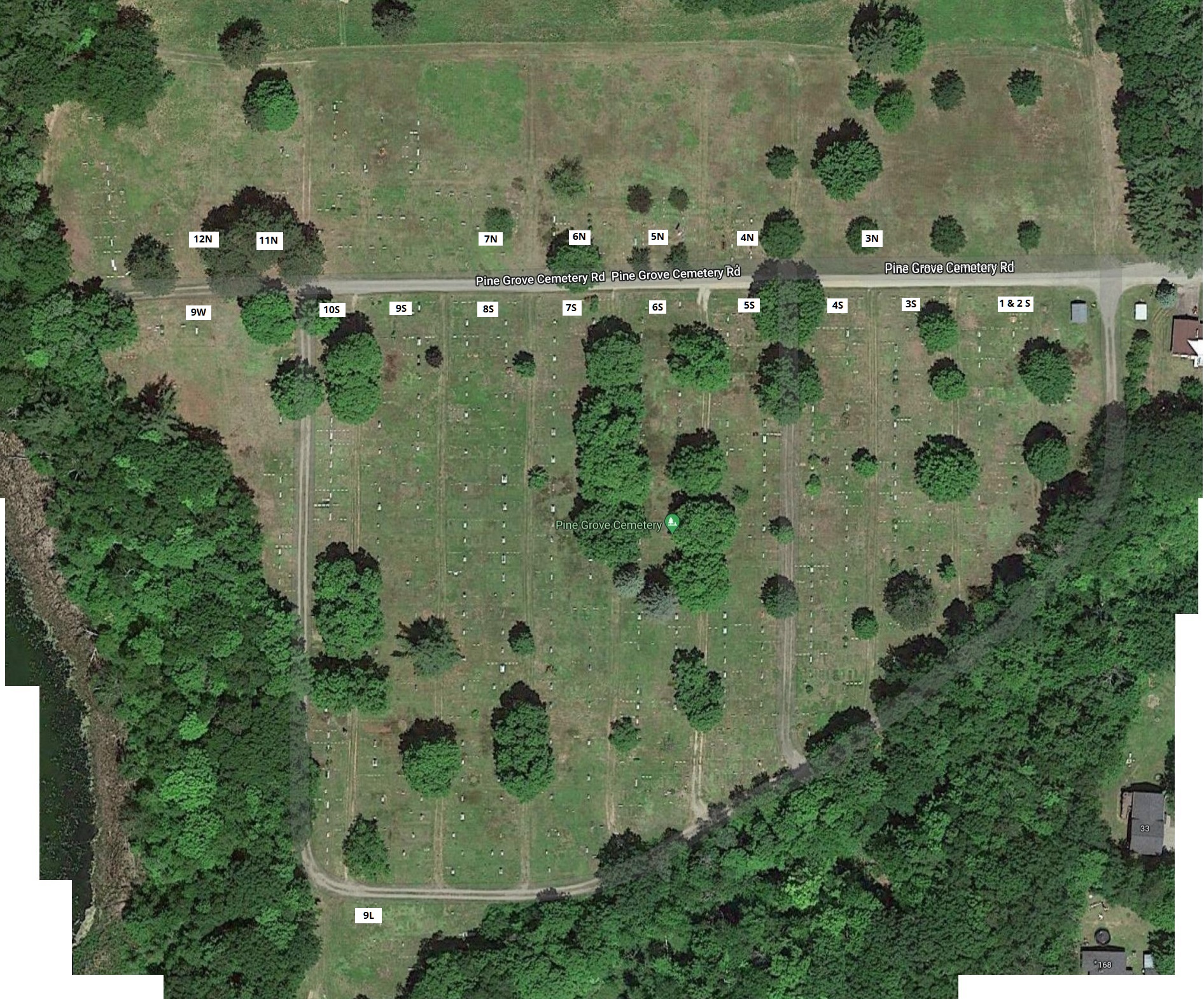The image is an aerial or satellite photograph of Pine Grove Cemetery. It showcases a well-manicured cemetery with numerous plots, identifiable by white rectangles with numbers such as 12N, 11N, 9W, 75, 85, 55, and 45. The primary road, Pine Grove Cemetery Road, runs through the upper-middle section of the photograph and branches off into smaller roads providing access to the various plots and headstones. Dense green grass covers the ground, complemented by multiple shades of lush green trees surrounding and scattered within the cemetery. Additionally, on the right side of the image, there are houses with brown and grey roofs, while dark green, more densely treed areas appear on the left side, adding to the serene landscape.